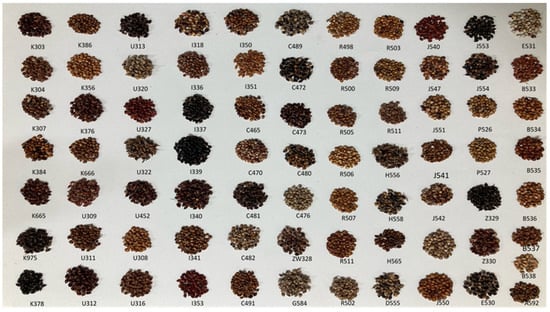This image features a meticulously organized display of seeds carefully categorized by type, color, and coded identifiers. Arranged in seven vertical columns and eleven horizontal rows, each small circular pile of seeds is distinct in hue and shape. The colors of the seeds vary widely, including shades of black, red, brown, light brown, cream, blue, pink, green, and purple. Over a hundred piles are presented on a white or light gray background, with each pile labeled by a code comprised of a letter followed by three numbers. This systematic layout likely aims to catalog the diversity of seeds, with the black-inked codes serving as identifiers for each type.